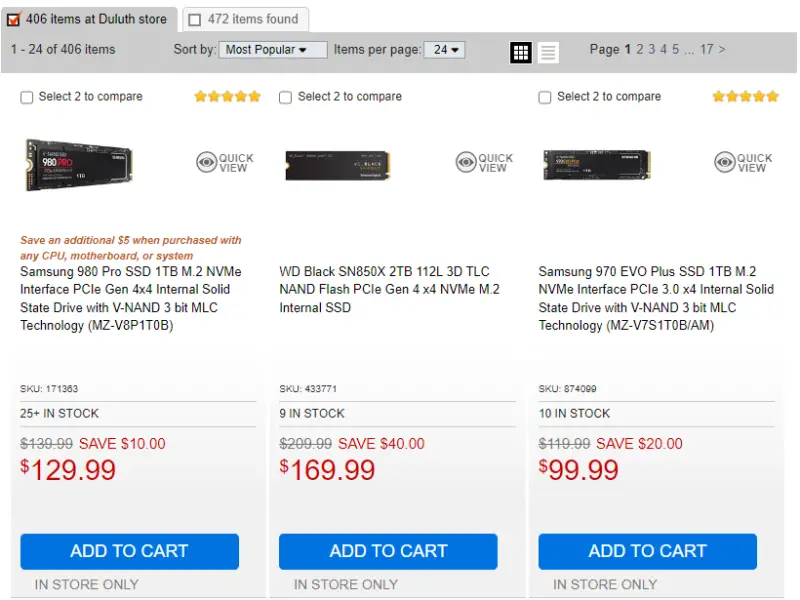The image showcases a website dedicated to selling computer parts. In the upper right corner, there is a noticeable white checkbox outlined in black with a red checkmark, signaling "406 items at the booth store." The navigation options include sorting by "Most Popular," displaying "24 items per page," and currently showing "Page 1."

Below this navigation bar, there are several computer components on display. The leftmost product is highlighted by a promotional message: "Save an additional $5 when purchased with any CPU, motherboard, or system." This product is a Samsung 980 Pro SSD, featuring a 1TB capacity, M.2 form factor, NVMe Interface, PCIe Generation 4.4, and V-NAND 3-Bit MLC Technology. Priced at $129.99, it has a rectangular black design.

In the center, the product is a WD Black SN850X SSD boasting a 2TB capacity, 112L 3D TLC NAND Flash, PCIe Gen 4x4 NVMe M.2 Interface. Also rectangular and black, this SSD is listed at $169.99.

The rightmost product is another internal drive, the Samsung 970 EVO Plus SSD, featuring a 1TB capacity, M.2 form factor, NVMe Interface, PCIe 3x4, and V-NAND 3-Bit MLC Technology, priced at $99.99.

Each product listing includes a blue "Add to Cart" button with white text, simplifying the purchasing process for shoppers.